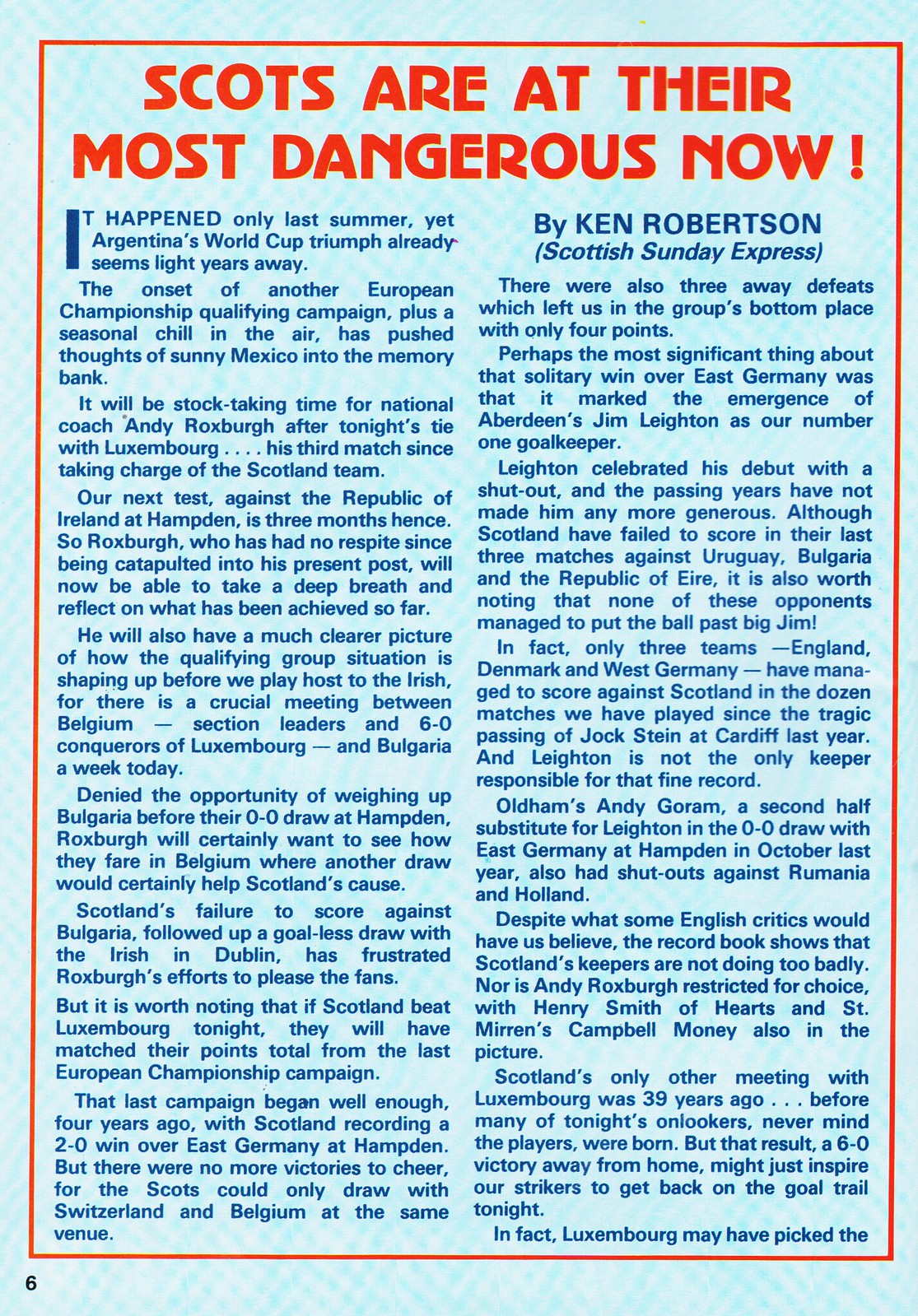This is an image of page six from a print soccer publication. The page features a light blue background with an orange border encircling it. The article's title, "Scots Are At Their Most Dangerous Now!" is prominently displayed in large, bold, orange font at the top center of the page. Written by Ken Robertson, with the attribution "Scottish Sunday Express" in italics, the text is presented in two columns of darker blue print. The opening paragraph starts on the top left and reads: "It happened only last summer, yet Argentina's World Cup triumph already seems light years away." The page number '6' is printed in black on the bottom left. The article discusses various countries, focusing on Argentina and the ongoing World Cup narrative.